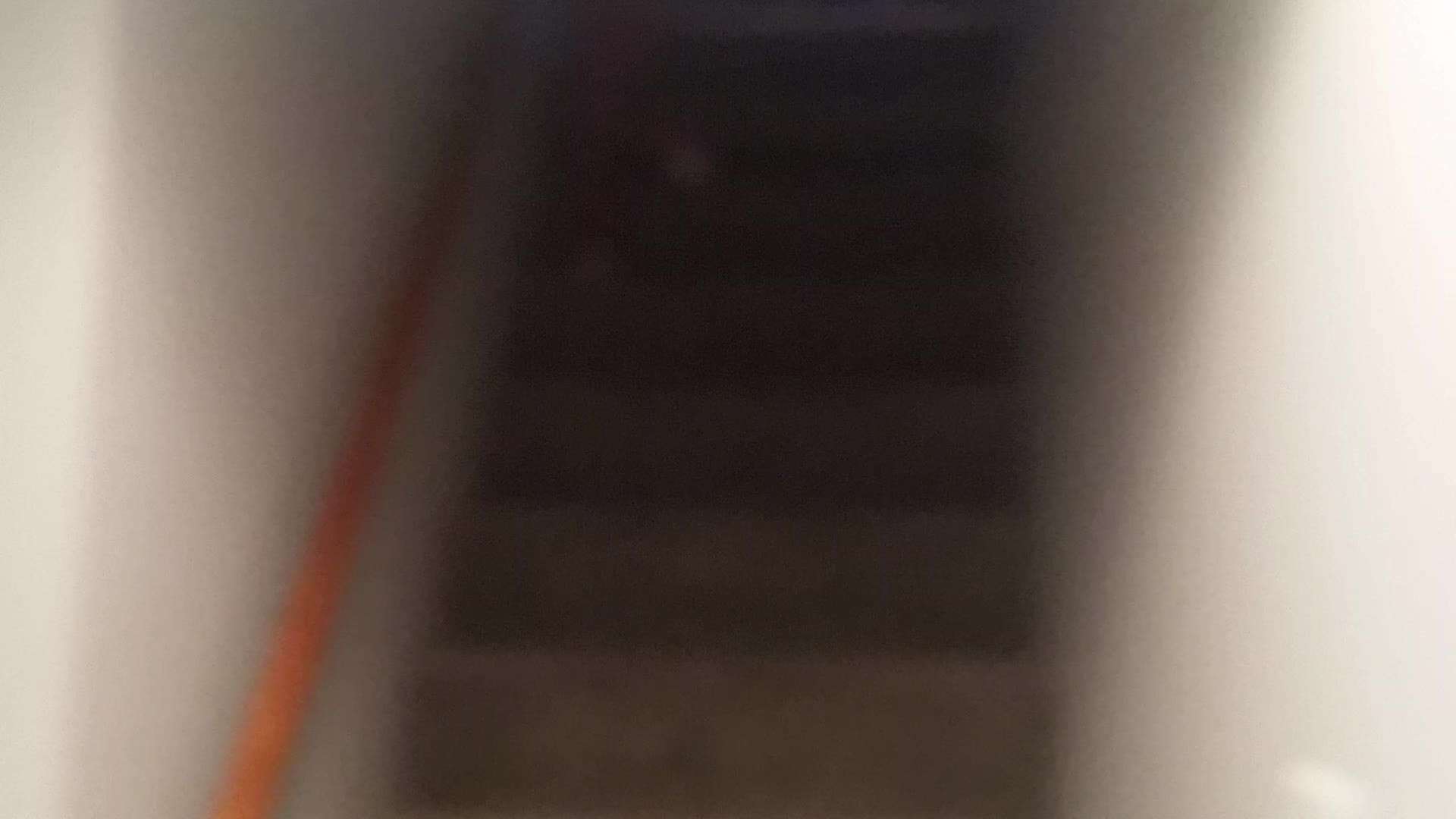The image depicts a stairwell with a distinctive hazy, low-quality texture, reminiscent of looking through a steamy mirror. Both walls on the right and left are painted white, and shadows are faintly discernible. The stairwell, positioned centrally, features stairs that appear to be concrete with a brown to light gray hue and some darker stains. An orange or red wooden handrail runs up the left side of the stairs. At the top of the steps, on the left-hand side, the indistinct legs of a person in red pants and white shoes are faintly visible, suggesting the person is mid-step, ascending the staircase. The lighting changes subtly from a brighter bottom right to a darker upper portion of the walls, adding to the overall hazy and blurry effect of the photograph.